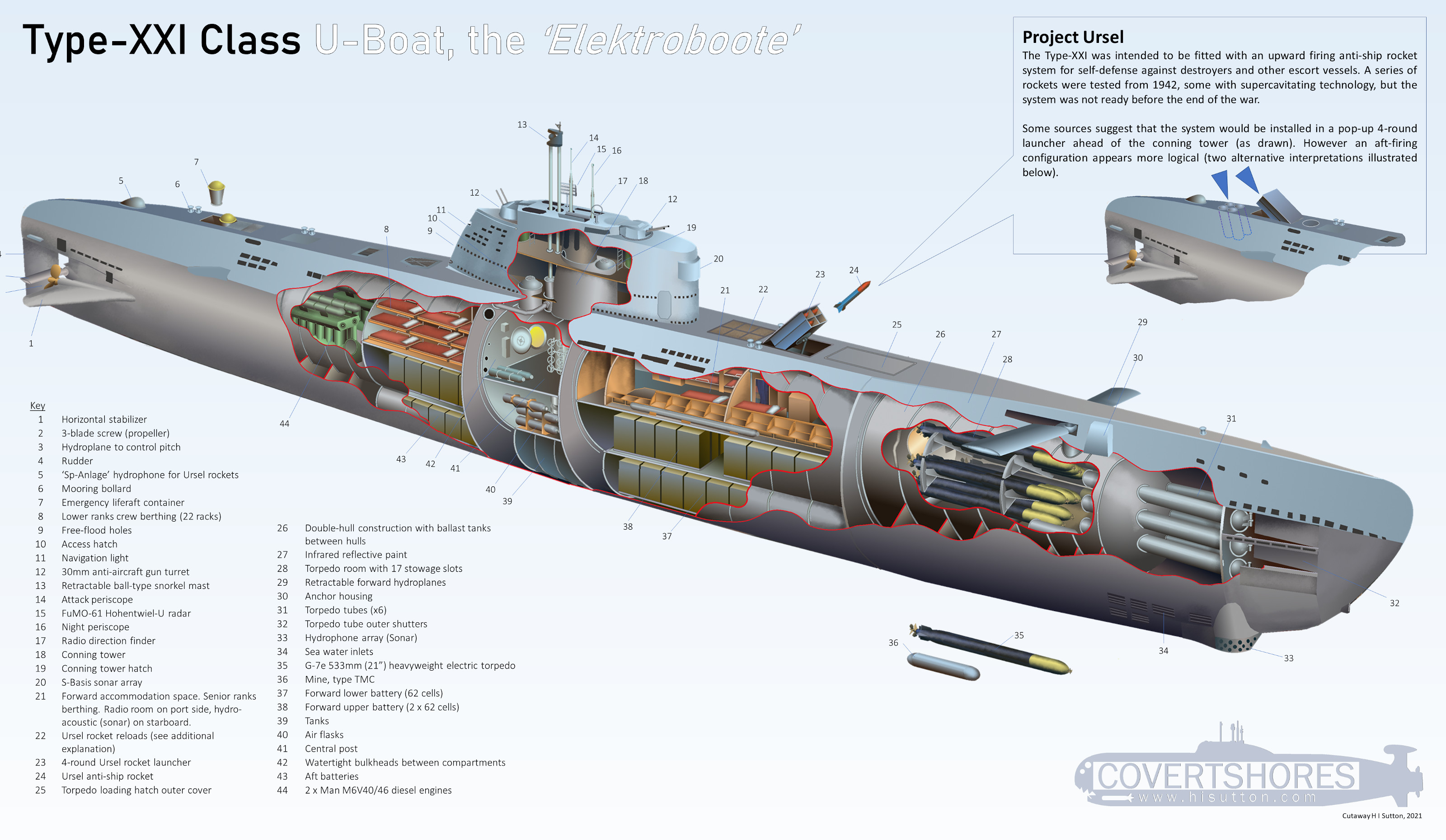The image is a detailed, graphic visual art piece depicting a Type-XXI Class U-Boat, known as the Elektroboote. The artwork is rectangular and features a cross-section view of the submarine, showcasing its inner compartments and structures. On a light blue background, the top left corner reads "Type-XXI Class U-Boat - Elektroboote" in bold lettering. The submarine's exterior is rendered in a sleek silver color.

In the image, multiple numbers with arrows point to different sections of the submarine, corresponding to a detailed legend that identifies each part. The visualization reveals various internal components such as torpedoes, sleeping quarters, the periscope, air tanks, and other crucial elements of the U-boat’s architecture. Notably, there is a highlighted section labeled "Project Ursel," providing an in-depth explanation of a specific weapon system located on the deck. Additionally, the phrase "Covent Shores" is artistically inscribed at the bottom right of the image, adding an extra layer of detail. Icons and labels are distributed throughout, particularly concentrated in the bottom left corner. The comprehensive and intricate depiction offers an insightful look into the sophisticated design of the Type-XXI Class U-Boat.